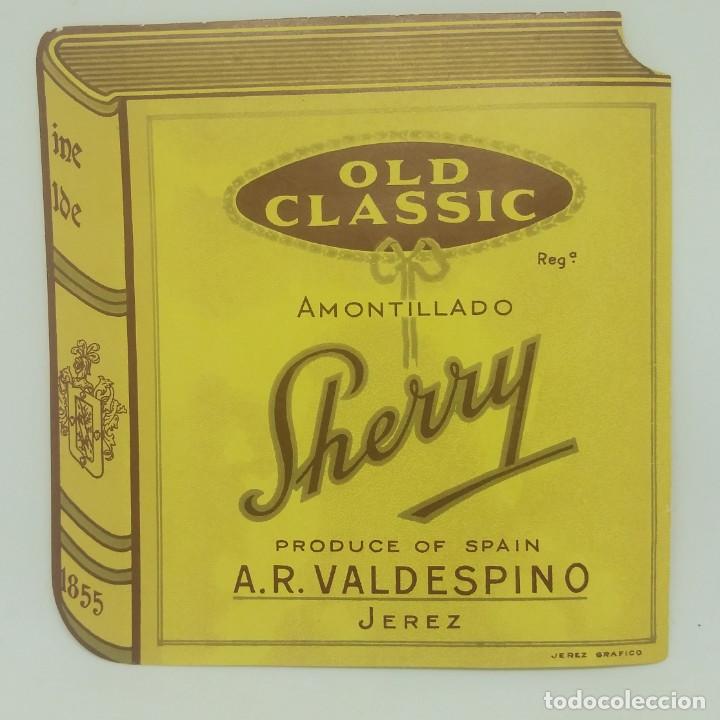The image features a detailed, almost cartoonish hand-drawn rendering of a thick yellow hardcover book with brown writing and intricate details. The book, set against a solid medium gray background, prominently displays its front cover, back binding, and top pages. On the front cover, within an oblong circular badge, is the title "Old Classic" in yellow, accompanied by a ribbon with a bow at the bottom. Below the bow, in small thin letters, is the word "Amontillado," followed by the large, diagonal cursive text "Sherry." Further down, in smaller brown letters, it states "Produce of Spain," and below that, in capital letters, "A.R.Valdespino" with a horizontal line separating it from the word "Jerez" underneath. 

On the back binding, the top features the word "Ineide" in an old-timey medieval font. The middle showcases a family crest adorned with flowers, and at the bottom, the year "1855" is inscribed. The book's mustard-yellow hue contrasts with its predominantly brown text and decorations. Overall, the book dominates the image, with only small portions of the gray background visible, and a white Spanish phrase "todo coleccion" appears in the bottom right corner.